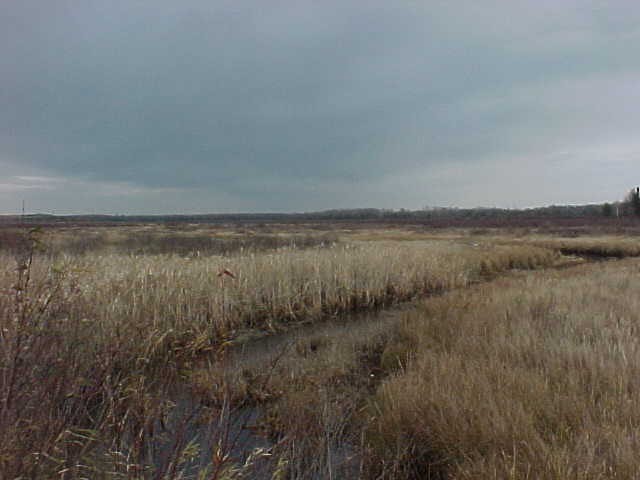The image captures a serene outdoor scene of a marsh area, likely just outside a town. The expansive field is dominated by tall grasses and weeds, many of which have a light brown, yellowish hue that suggests they might be dried or dead. Flowing through the foreground is a small stream or creek, cutting a narrow path through the overgrown vegetation, making the scene appear murky and swampy. The horizon is lined with various trees, including a distinctive cluster of pine trees to the far right. The sky above is mostly covered with an array of gray clouds, ranging from dark and brooding to lighter shades, hinting at an impending rainfall. Despite the overcast sky, there's a subtle indication that the photo was taken during the daytime, likely in the evening hours, as suggested by the quality of the light. The distant background shows faint outlines of mountains, adding a sense of depth to the landscape.